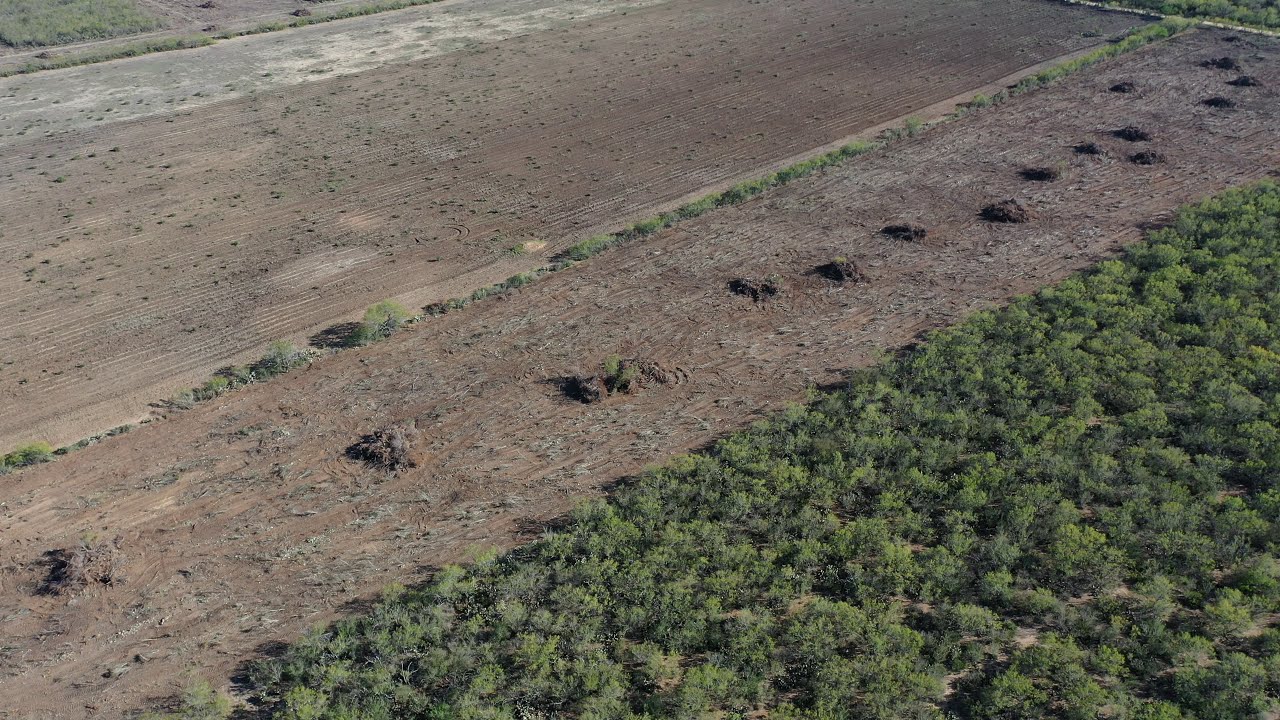The image captures an aerial view, likely taken by a drone on a sunny day, showcasing a series of empty crop fields. Dominating the lower right corner is a lush, dense area of green bushes, contrasting vividly with the barren expanses surrounding it. The green foliage stretches diagonally across this corner, bordered by what appears to be a drainage ditch. To the left of this green section lies a field characterized by brown dirt with some visible mounds, possibly gopher holes. Moving further to the left, the dirt continues, and clearly discernible within this stretch are subtle pathways and rake lines indicative of a recently sown field. Towards the bottom center of the image, there are patches of dirt showing signs of previous cultivation but currently barren, accentuated with rough patches and uprooted holes. This detailed depiction emphasizes the contrasts between the uncultivated green bushes and the largely empty, sunlit crop areas now devoid of any active farming.